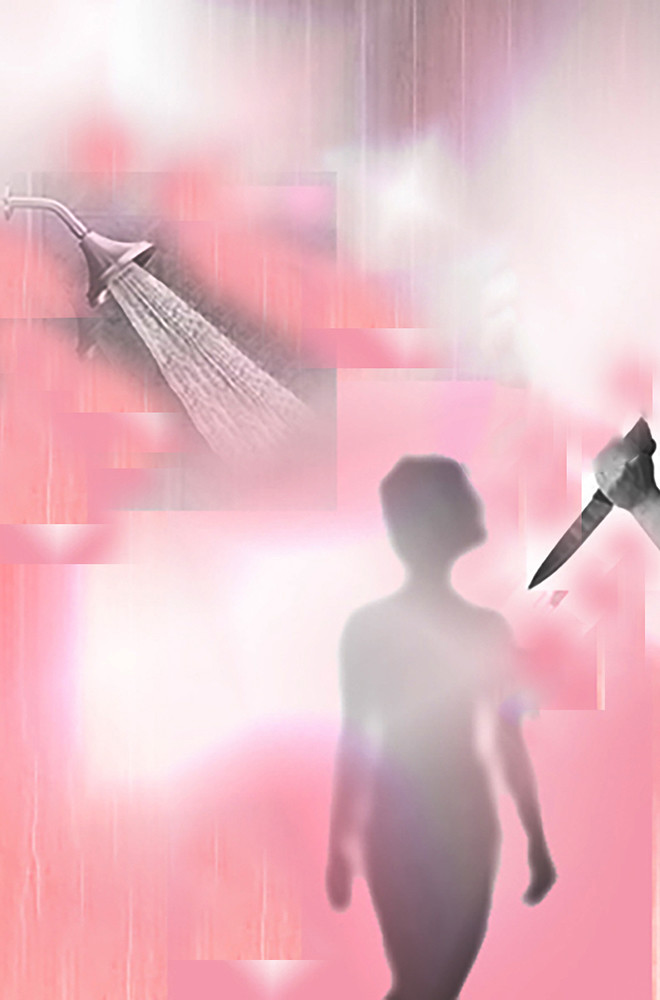In this digitally designed, artsy image, we see a spooky scene reminiscent of a classic horror moment. The rectangular artwork features a misty background comprised of varying shades of pink, hot pink, and occasional white splotches, giving it an eerie, glitchy appearance. On the upper left, a silver shower head sprays water fan-shaped downward, casting a shadow over a shower curtain and rod. Towards the bottom right, the silhouette of a feminine figure with short hair, a small waist, and wider hips stands, seemingly unaware of the looming danger. On the far right, a sinister hand gripping a large dagger is poised in a stabbing motion aimed at the figure. The unsettling use of red and black shadows adds to the dramatic tension, capturing a scene strikingly similar to the unforgettable shower scene from the movie "Psycho."